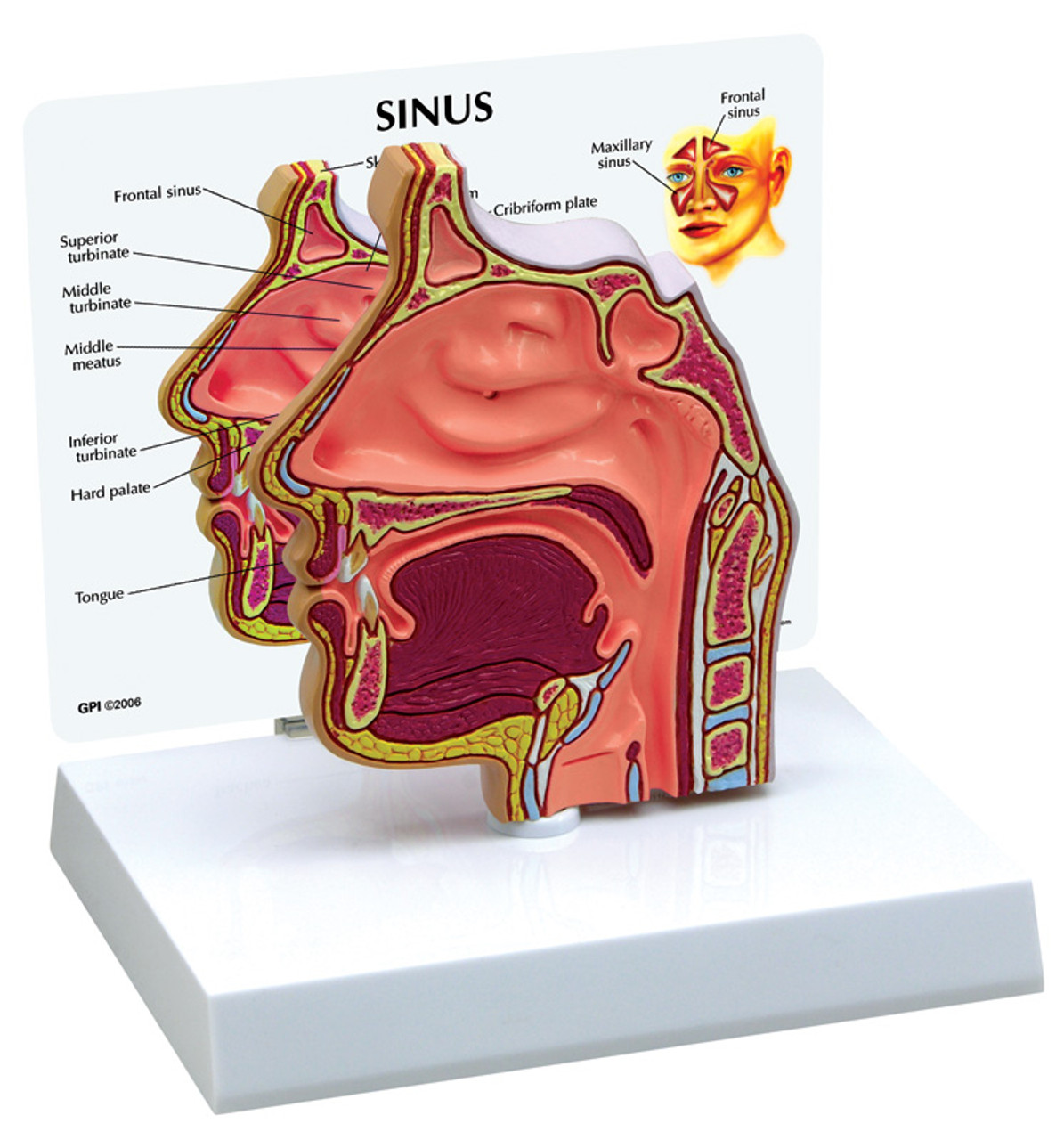The image is a detailed educational diagram of the anatomy inside the head, focusing on the sinuses. It is displayed on a white rectangular stand with a white background. At the top, in prominent black text, it reads "sinus." The sculpture is a cutout view of the front portion of a face, revealing the internal structures, including the mouth, nose, and various sinuses. An accompanying labeled image enhances the sculpture, pointing out specific parts such as the frontal and maxillary sinuses, turbinates, middle meatus, hard palate, and tongue. The diagram is slightly diagonal, with arrows indicating different sections and their names. The visual representation includes colored sections like pink tissue and purple areas to differentiate between structures, providing a comprehensive educational overview of the nasal and oral cavities in a cross-sectional format.